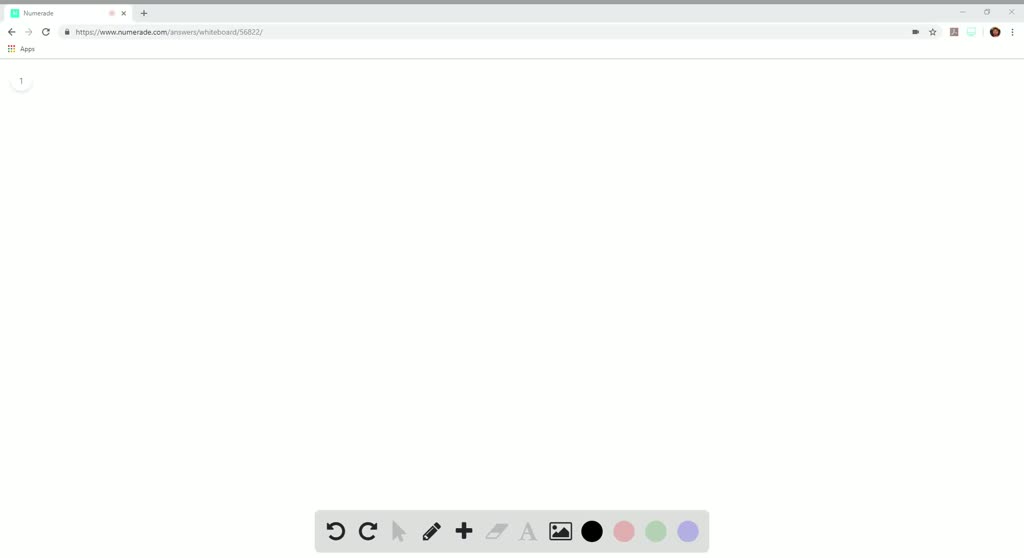This image is a detailed screenshot of a website interface. At the very top, a gray bar displays the website's name, which begins with an "N," although the text is too small to be legible. Directly below this, the standard web browser elements appear: a back button, a refresh button, and a gray address bar where users can type in the desired URL. To the right of the address bar, there is a small user avatar and a button for additional features.

Further down, a section labeled "apps" indicates that this screen is intended to display a collection of applications available to the user. However, the space appears empty, suggesting that the user either has not set up any apps yet or does not utilize this feature.

At the bottom of the screen, a compact sub-menu provides quick access to common functions such as backward and forward navigation and includes an icon resembling a pencil, likely for editing purposes. This screenshot captures the structure and navigation elements of the website but lacks detailed content visibility.